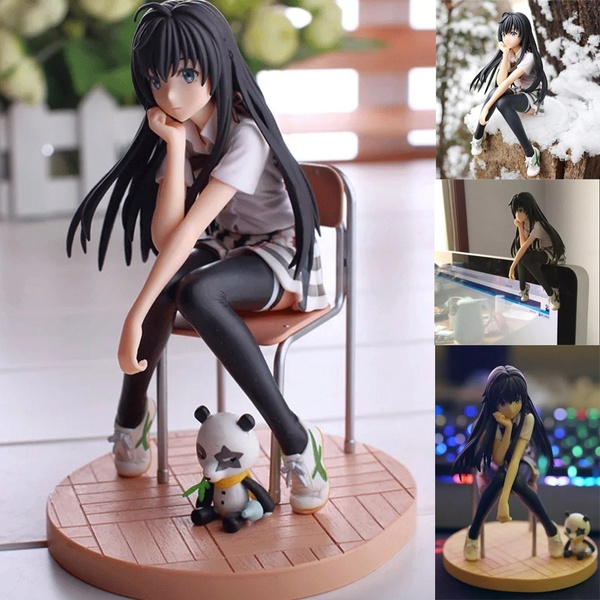This is a detailed color photograph showcasing an intricately designed three-dimensional figurine of a young anime-styled woman, seemingly made from a smooth, clay-like material. The main scene features the figurine seated on a copper-colored school chair with her feet apart and knees together, giving off a slightly contemplative or bored demeanor. She has long, dark, motion-styled hair, wears a short-sleeved white shirt, a plaid skirt, and black leggings with white stripes at the top. Her right hand supports her chin with the elbow resting on her knee, while her left arm extends down between her knees, resting over her lap. She completes the look with white sneakers adorned with green cross logos on the sides. Positioned at her feet is a small panda bear with a yellow handkerchief around its neck and a distinctive black star over its left eye, evoking a playful, mascot-like presence.

Additionally, this primary image is accompanied by three smaller views of the figurine. One shows her seated on a snow-topped brick, another perched on a computer monitor, and the last one offers a detailed front perspective of the figurine along with her panda companion. The entire setup rests on a small round platform styled to resemble a parquet floor, adding to the overall charm and intricate detail of the scene.